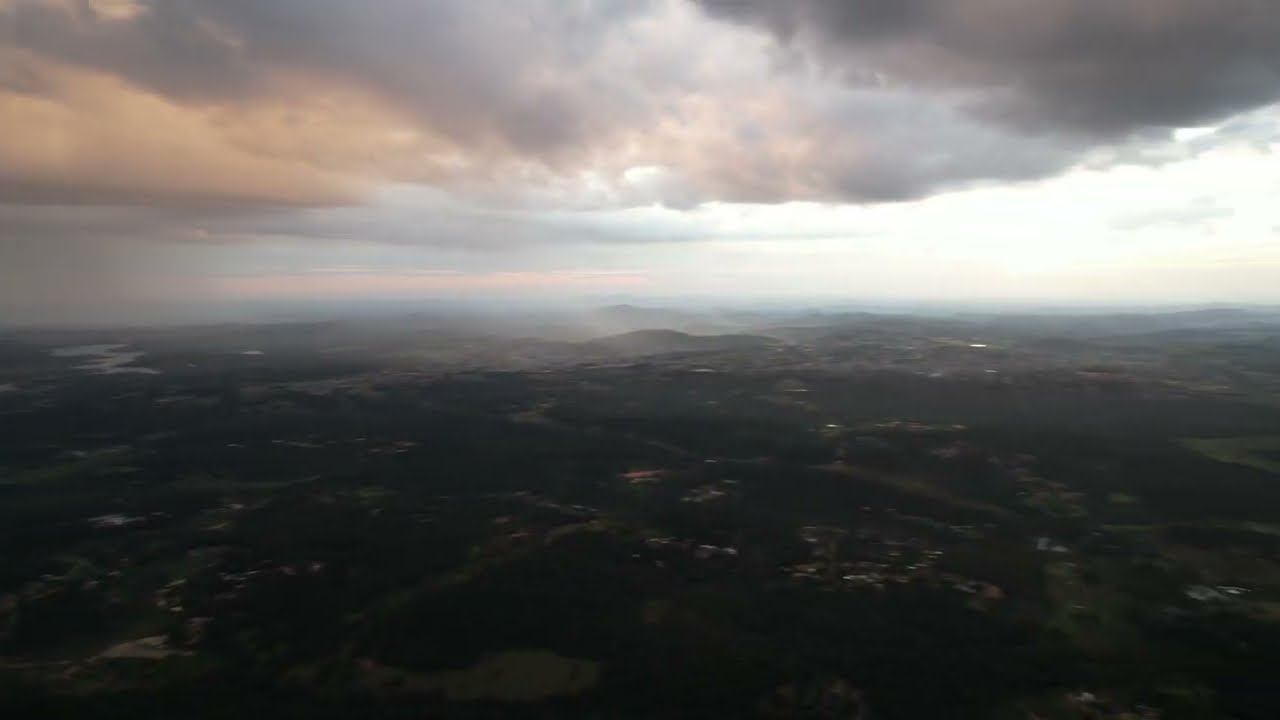This atmospheric, full-color aerial photograph captures a sprawling landscape under very low lighting conditions, likely during dawn or dusk. The top portion of the image is dominated by thick, fluffy clouds in varying shades of dark gray and pinkish-orange, indicative of heavy overcast skies with potential rain. A thin stream of light penetrates through a break in the clouds, casting a faint glow over the scene. Beneath this dramatic sky, the ground below is largely obscured and blurred, with hints of green hills and a scattering of indistinct, rectangular rooftops suggesting a suburban or rural area. Along the horizon line, faint outlines of mountains are visible, adding depth to the composition. On the far left, there is a barely discernible, winding river or small body of water, adding a subtle but significant feature to the landscape.